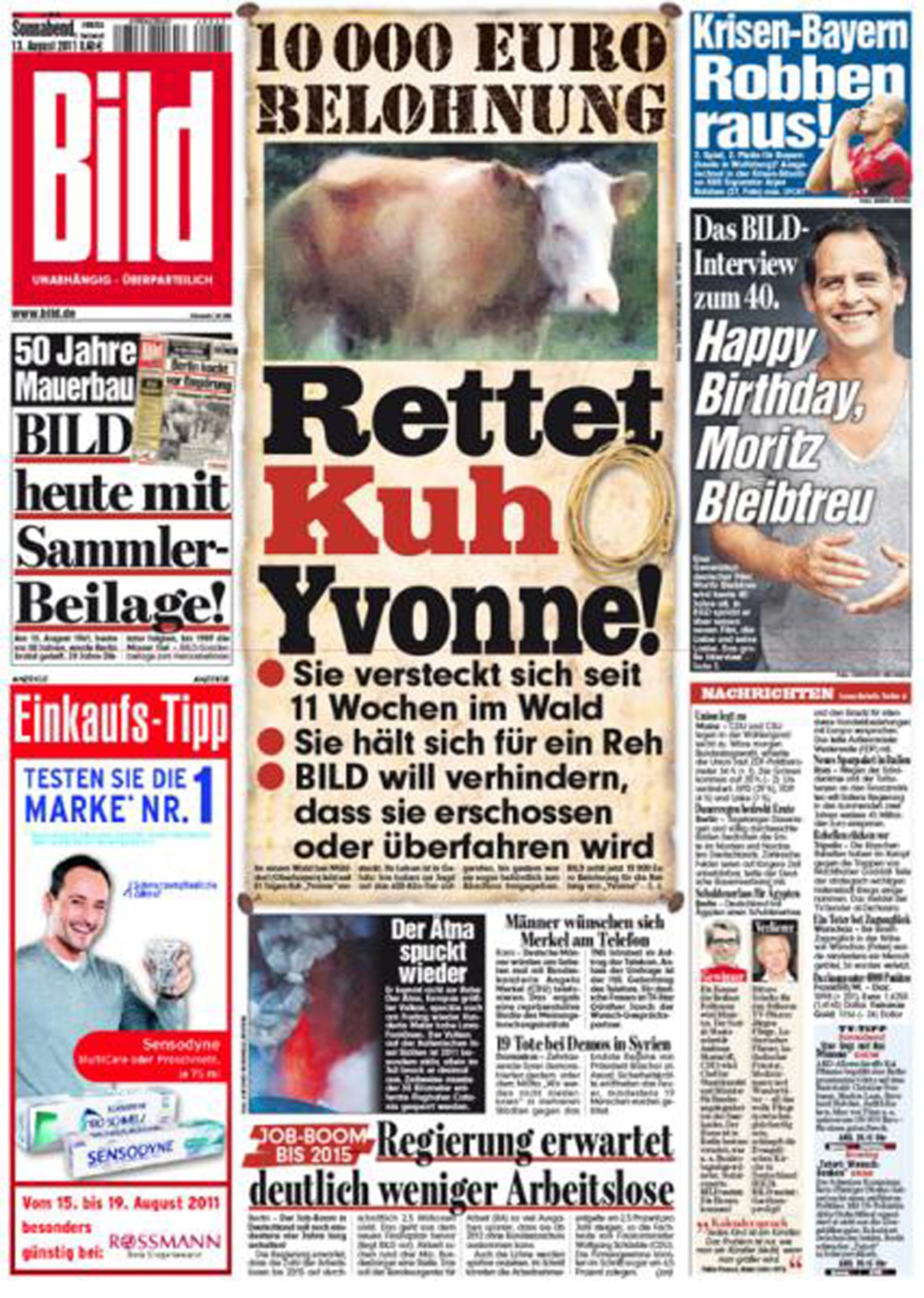The image is a portrait-oriented scan of the front page of a German tabloid newspaper, likely BILD, suggested by its distinctive red rectangular logo in the upper left corner, with elongated white letters "BILD". A barcode is positioned above the logo, featuring various thick and thin black vertical lines tightly packed together. The page is divided into three vertical columns, the middle one being wider than the two outer ones. 

Prominently displayed in the top center is a bold headline offering €10,000, possibly related to capturing a cow, which is shown in a photograph below the headline. The cow is brown with a white head. Next to this, at the bottom center of the page, is an image of smoke and flames, suggesting a story about a fire or volcano eruption.

On the upper right-hand side, there is a photo of a footballer, indicating sports coverage. Below that, a smiling man in a gray T-shirt is featured with the text "Happy Birthday," celebrating his turning 40. 

The bottom left corner contains an advertisement for Sensodyne toothpaste, and another ad for Rolex is visible nearby. Due to blurring in the bottom right half of the image, additional smaller headlines and texts are unreadable. The numerous articles and photographs scattered across the page, in a language perceived to be German, contribute to the cluttered yet lively layout customary for a tabloid newspaper.